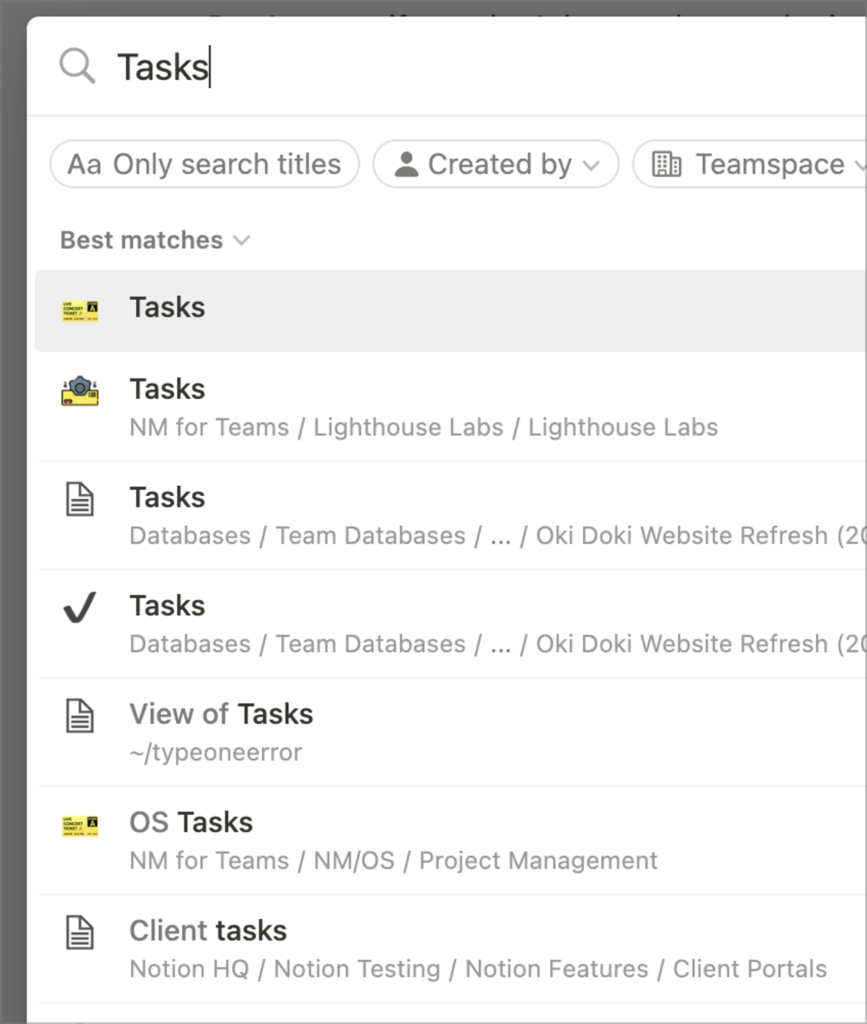In the image, a pop-up window with a light gray background and black text is displayed. The main feature is a search bar where the user is currently typing the word "tasks." To the left of the search bar, there's a magnifying glass icon. Below the search bar, there are various filter buttons, including one labeled "Search only titles created by TeamSpace," which is accompanied by a matching icon to its left.

Additionally, there's a drop-down menu labeled "Best matches" to further refine the search results. The results are listed below the search bar, showcasing a series of tasks. Some of the entries read: "Tasks, task nm for team/lighthouse labs/lighthouse labs," "Tasks, databases/team databases/…" followed by "okie dokie website refresh (20…)," which is partially cut off on the right.

Other entries include "Tasks, databases team/team databases/…/okie dokie website refresh," "New types of tasks," "OS tasks," and "Client tasks." Each task entry is accompanied by accent or subtitle text that likely provides additional context or categorization, possibly indicating the different levels of folders containing these tasks. However, the detailed meaning of these folder levels or categories is not immediately clear.